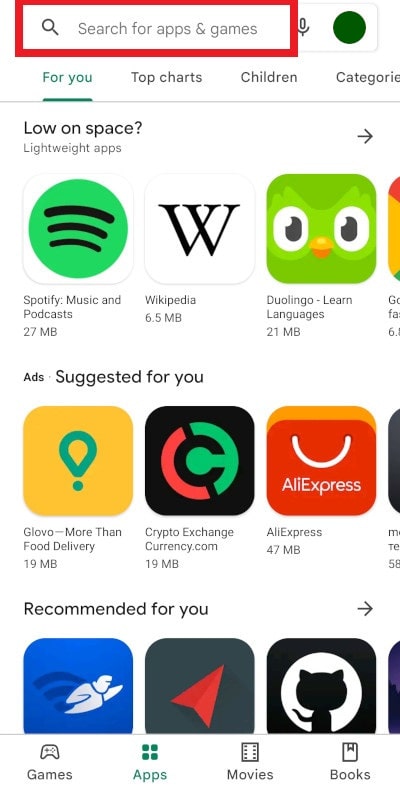This is a detailed screenshot of a Google Play Store page displayed on a smartphone. At the top of the screen, there's a prominently featured search bar with the placeholder text "Search for games and apps," highlighted with a red outline for emphasis. Beneath the search bar, a navigation menu lists the tabs "For You," "Top Charts," "Children," and "Categories." The "For You" tab is highlighted in green and underlined, while the other tabs are depicted in dark grey. A grey divider line separates the navigation menu from the content below.

Next, there's a notification area that reads “Low on space?” followed by a suggestion for "Lightweight apps" with a forward arrow icon on the right side indicating additional navigation options. A row of popular app icons is showcased below, including Spotify, Wikipedia, and Duolingo.

Further down, there's a section titled "Ads: Suggested for you" featuring advertisements for various services like "Glovo - More Than Food Delivery," "Crypto Exchange - Currency.com," and "Aliexpress." Finally, a "Recommended for You" section is visible with a clean, white background, suggesting more personalized app recommendations based on the user's interests.